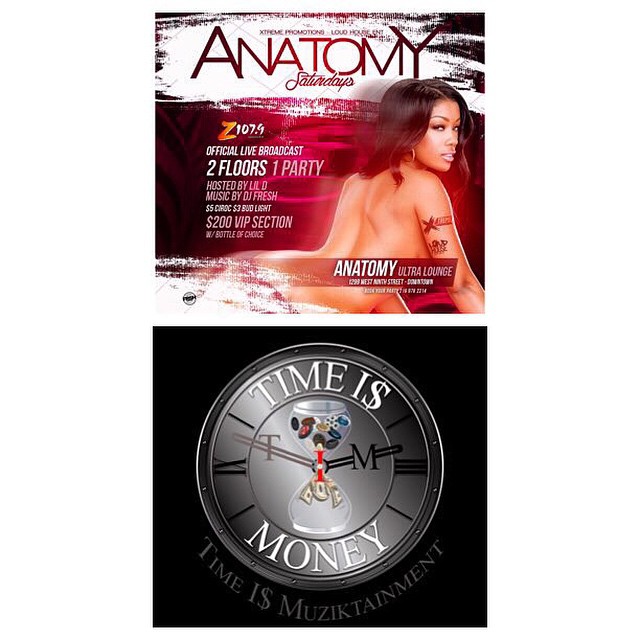The advertisement image is split into two distinct sections. The top section promotes "Anatomy Saturdays" at the Anatomy Ultra Lounge, featuring a Z107.9 official live broadcast. The headline "Anatomy Saturdays" is displayed against a white background with a paintbrush stroke effect, followed by event details, including "Two Floors, One Party" hosted by Lil D, with music by DJ Fresh. It also mentions a $200 VIP section. A nude black female, looking back seductively, occupies the right side of this section. She has tattoos on her right tricep and is adorned with earrings, with "Anatomy Ultra Lounge" text partially overlaying her image.

The bottom section of the image contrasts with a black background featuring a sleek silver clock face with Roman numerals. Central to this section is an hourglass positioned on the clock, filtering buttons or chips into dollar signs, emphasizing the theme "Time is Money." The phrase "Time Is" is inscribed at the top, with the "S" stylized as a dollar sign, and "Money" at the bottom. Beneath this visual, the text reads "Time is Musictainment," stylized as "M-U-Z-I-K-T-A-I-N-M-E-N-T." The clock face has white markings and black hands, reinforcing the message that aligns time with both money and music entertainment.